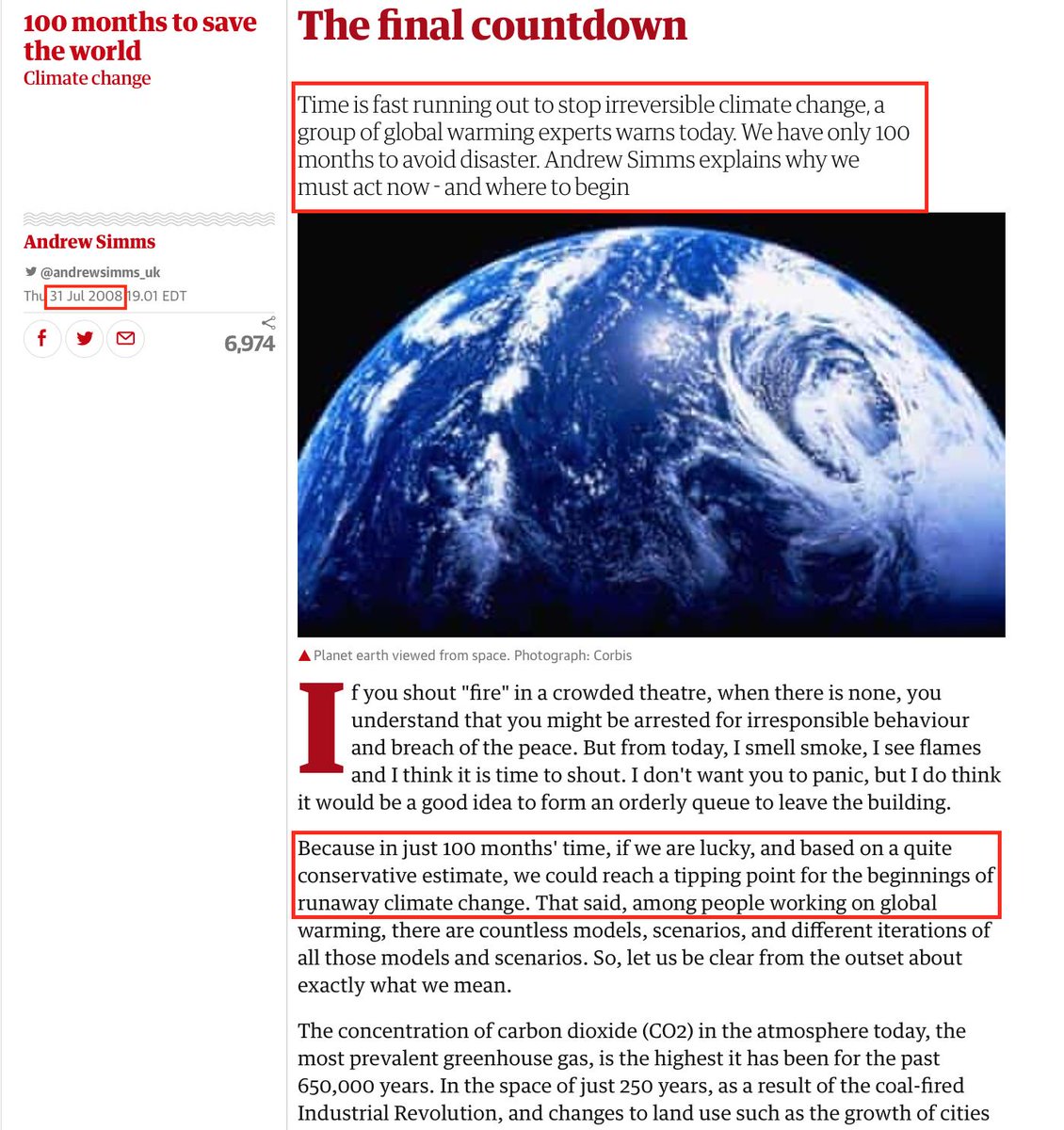The image depicts an article titled "The Final Countdown" in darkish red font, with only the "T" capitalized. On the left side of the article, in slightly lighter red, the phrase "100 Months to Save the World" is prominently displayed, followed by "Climate Change" with both words capitalized. Below some blank white space, a line separates this section from the author's name, "Andrew Simms," in roughly the same red color, with a Twitter handle "@AndrewSimms_UK" underneath it. The article's date, "31-JUL-2008," formatted in UK style, is marked with a red box and is accompanied by the time "19:01 EDT." Additionally, two sections of the text are highlighted with red boxes: the first paragraph and part of the third paragraph. A striking blue image of Earth, with white clouds, is placed below the first paragraph, while a vivid red eye is featured in the second paragraph.